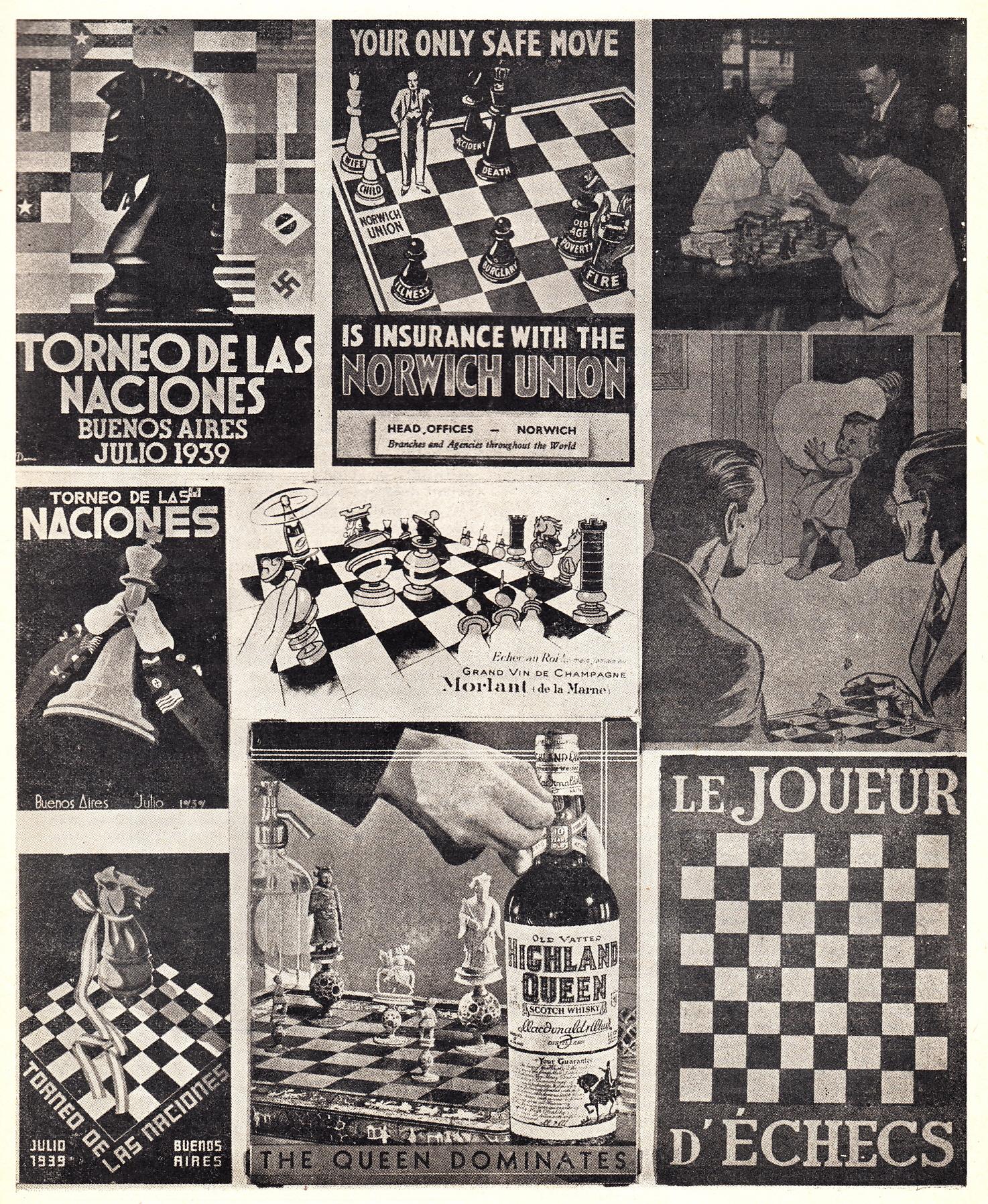This black-and-white advertisement from 1939 is centered around the theme of chess and insurance. The top left corner features an image of a black knight chess piece, overlaying a background filled with various countries' flags. Below this, in a black box with white letters, it reads "Torneo de las Naciones, Buenos Aires, Julio, 1939." Adjacent to the knight piece is an evocative collage, including a chess board inscribed with "Norwich Union" and cautionary words such as "old age," "poverty," and "fire" at the base of different chess pieces. Above this inscription, a caption proclaims, "Your Only Safe Move," emphasizing the importance of insurance with Norwich Union. To the right, a mixture of photographs and cartoons captures the world of chess: men engrossed in a game, another chess board beneath a wine bottle, and a scene with a little boy carrying a lightbulb into a room where two people play chess. Dominating the scene is a raised king chess piece, symbolizing strategic thinking. The advertisement is peppered with text fragments such as "Le Jour," "Highland Queen," and “The Queen Dominates,” making it a rich, layered historical piece showcasing the convergence of chess and life insurance.